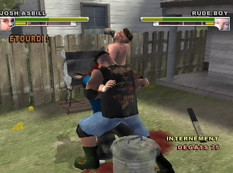This image is a detailed screenshot from an early 2000s 3D fighting video game. The scene takes place in a dingy backyard, partially enclosed by a rickety wooden picket fence. A barbeque grill, with a bare-chested person attending it, stands out in the background. The two main characters, Josh Asbill and Rude Boy, are engaged in a fierce fight depicted in the foreground. Josh appears to be in the process of throwing or grappling Rude Boy, who has slightly better health.

At the top of the screen, the status bars and avatars for the characters are displayed: Josh Asbill on the left with a green and yellow health bar at half capacity, and Rude Boy on the right with a health bar at about 75%. The game interface also includes the words "ETOUDI!" under Josh’s health bar and "INTERMENT DEGATS 75" at the bottom right of the screen, indicating game stats or actions, all presented in a non-English language. The ground is littered with environmental details such as blood pools, a grey metal trash can, and a machete-like object near the combatants. The overall graphics are polygonal and lack vibrant colors, giving the game a dated visual style.